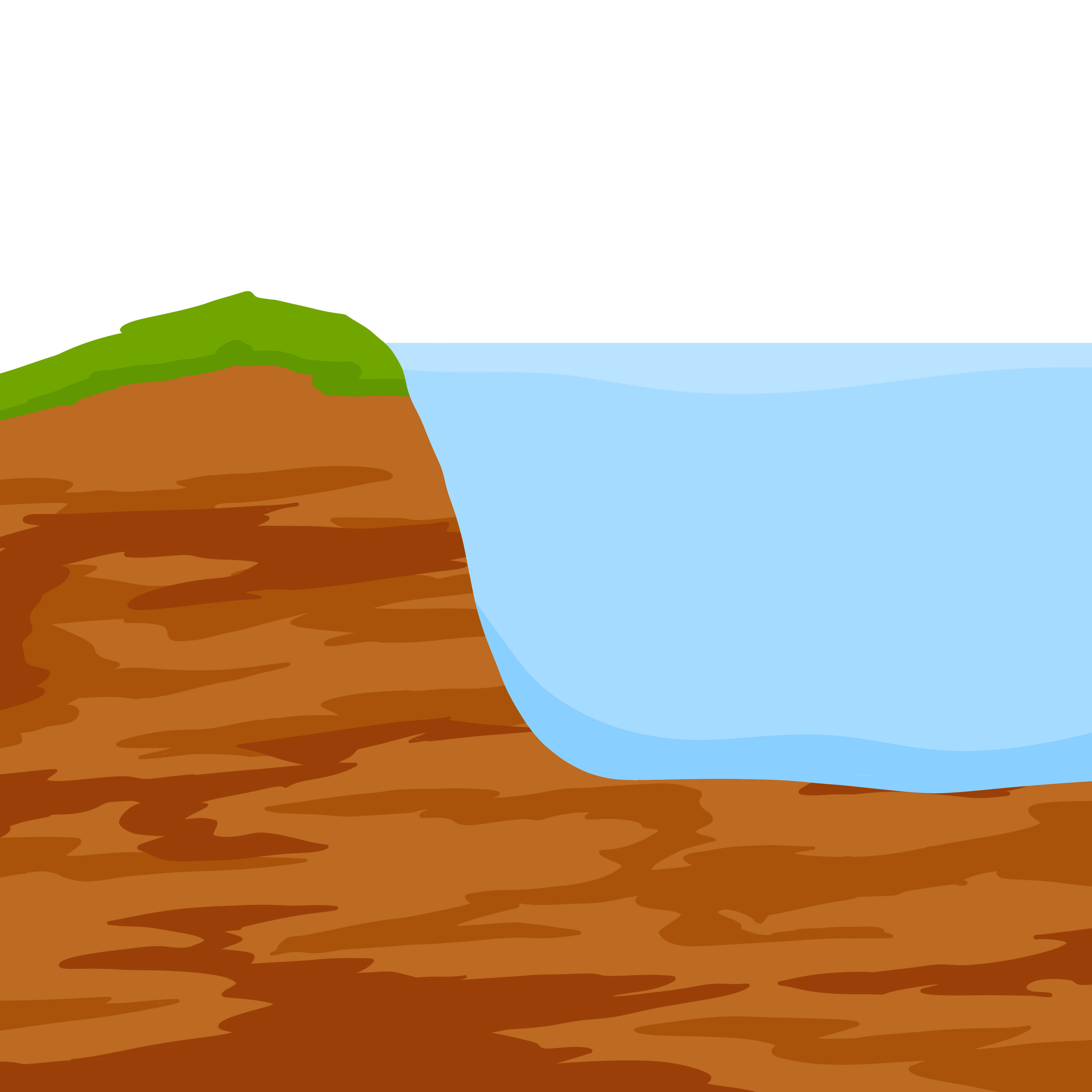This image is a very basic, simplistic illustration, likely drawn or rendered for educational purposes, depicting a river basin or embankment leading into a body of water. The illustration prominently features a large, L-shaped mound of earth that occupies roughly 85% of the image. This mound begins in the upper left corner, descends diagonally down towards the center, and then extends horizontally across the bottom.

On top of the mound is a patch of grass, characterized by its varying shades of green, with a darker green at the edges transitioning to a lighter green in the middle. The earth itself is depicted in three distinct shades of brown—light, medium, and dark—arranged in horizontal, wavy patterns to suggest stratified soil layers. These layers transition from light brown at the top to darker shades at the bottom, giving the mound a natural, realistic texture.

To the right of the mound lies the body of water, which forms the basin. The water is illustrated in a gradient of blues, starting with a pale light blue at the surface, deepening to medium blue in the middle, and finishing with a darker blue at the bottom, indicating depth. The water occupies most of the center-right portion of the image.

Overall, the colouring is bright and conspicuous, making the elements—grass, earth, and water—easily distinguishable. The top of the image is left pure white, enhancing the clarity and simplicity of the depiction.